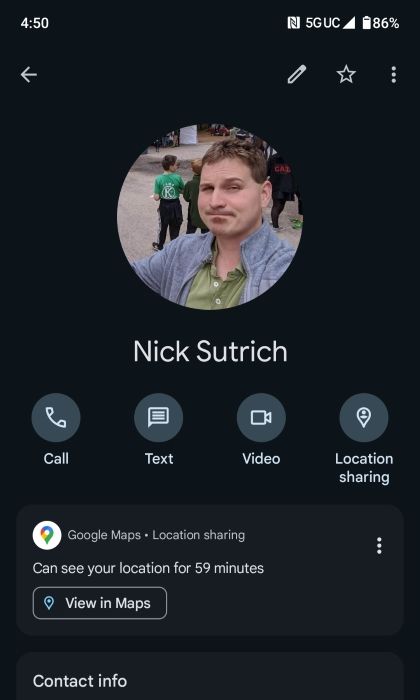In the top left corner of the image, the screen displays a signal strength of "450" along with a full 5G UC cellular connection, indicated by "5G UC." The battery icon shows an 86% charge, nearly full but a small part remains unfilled. 

The main focus of the image is a man named Nick Sutrích, characterized by his white skin, short brown hair, a mustache, and a slight goatee. Nick is dressed in a gray jacket over a green button-up shirt. His facial expression is notable for having one eyebrow raised and the other in a normal position. Behind Nick, there are several other people, suggesting a social or public setting.

Under Nick's name, several buttons are displayed including "Call," "Text," "Video," and "Share Location," each with corresponding icons: a phone, a text bubble, a webcam, and a location pin, respectively. Below these options is a section titled "Google Map location sharing," indicating that Nick's location can be tracked for 59 more minutes. To the right of this information, there is a section with three dots and a bubble that reads "View in the map." At the very bottom of the interface, contact options are provided, including a phone icon for calling, a text bubble for messaging, a camera for video calls, and a pinpoint icon for location sharing.